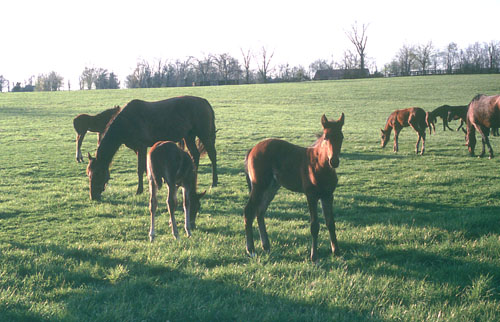In this picturesque image of a serene, emerald green meadow, several horses, predominantly with dark brown sable coats, graze contentedly. The scene is bathed in the warm light of the setting sun, which casts elongated shadows and creates a peaceful, pastoral atmosphere. In the background, amidst a slew of barren trees hinting at the winter season, a few farmhouse structures are visible, adding a rustic charm to the landscape.

At least seven to eight horses populate the field. Three of the closer ones, which have lighter brown legs, appear smaller and might be ponies. One of these, standing closer to the viewer, is illuminated by the sunlight and bears a distinguishing black mane. Another notable horse in the foreground looks directly at the camera, seeming curious about the observer. Most of the horses are engaged in grazing, with the two further back blending more into the shadowy backdrop.

Overall, the scene captures a tranquil moment in nature, highlighting the simple beauty of the horses against the lush green grass and the subtle intricacies of the interplay between light and shadow.